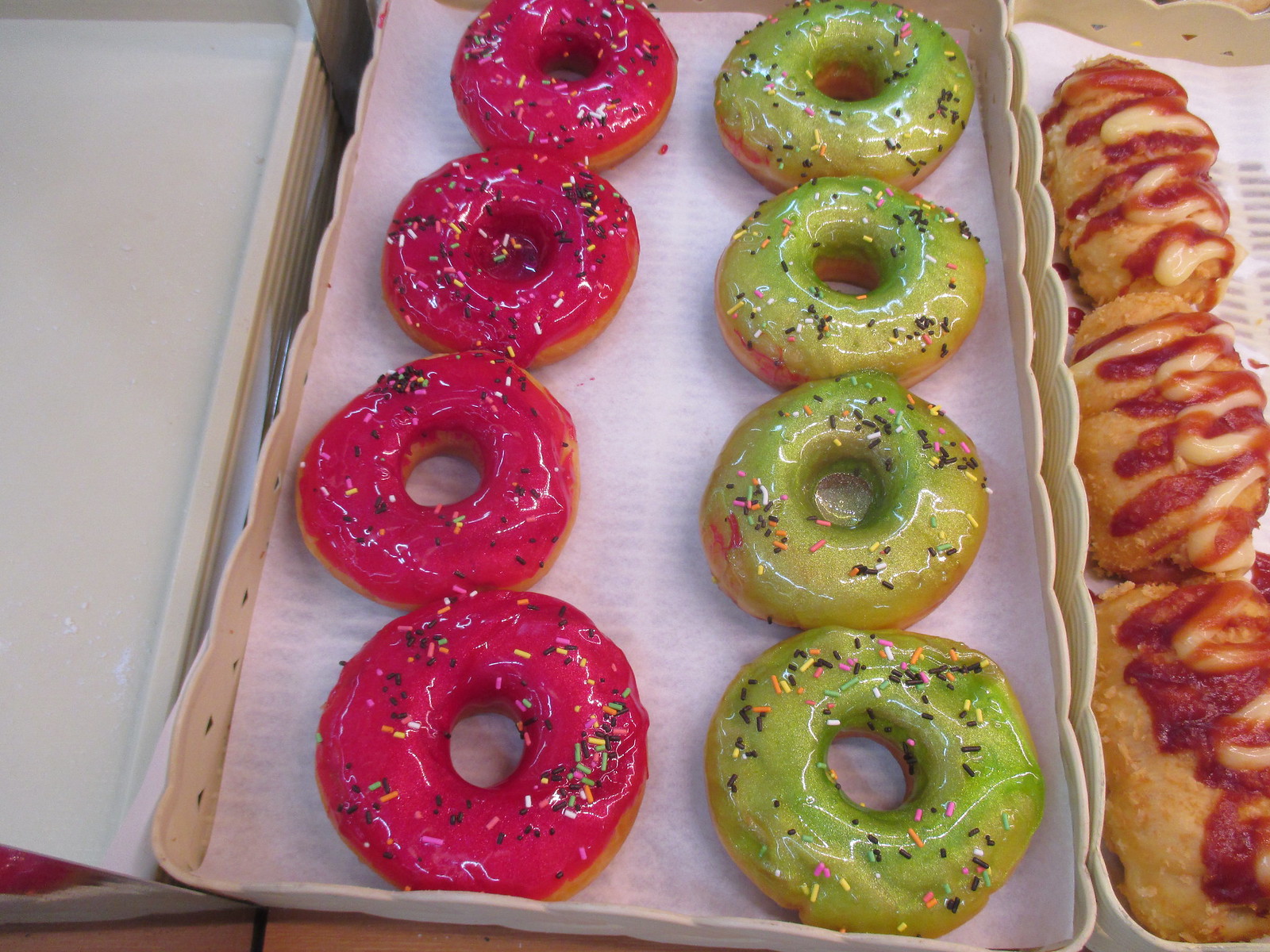The photograph showcases three trays arranged horizontally. On the left side, there's an empty white tray. The central tray, which is the primary focus of the image, holds eight doughnuts arranged in two vertical columns. The left column features four round doughnuts with bright pink frosting and multicolored sprinkles. The right column has four doughnuts with a pale lime green glaze, also topped with rainbow sprinkles. Beneath these doughnuts, the tray is lined with wax or parchment paper. To the right of the central tray, another similar white tray holds a few pastries; they appear to be golden brown and crusty, possibly drizzled with red and yellow frosting. The overall lighting of the image is somewhat dull, but the foreground is in focus, highlighting the vibrant colors of the doughnuts and pastries. The background, which includes a bit of the surface underneath that seems to have some brown tiling or wood, is slightly blurry.